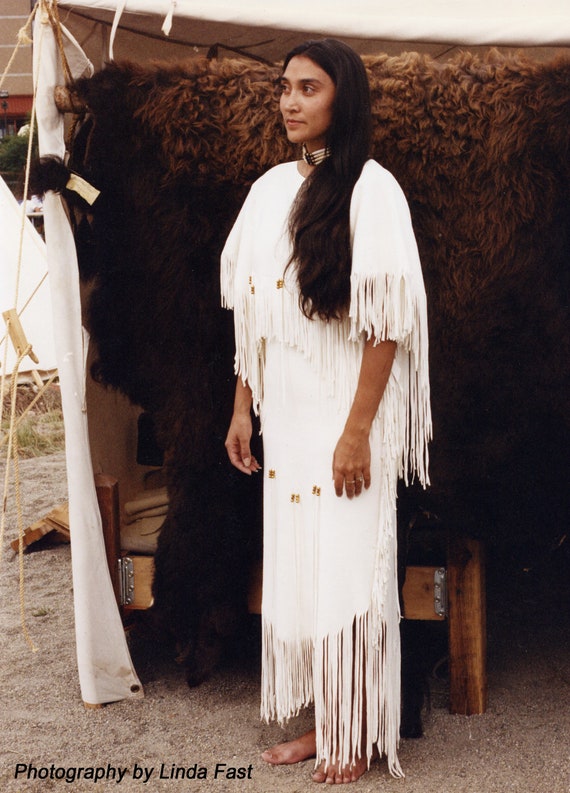This image captures a Native American woman standing barefoot on sand, facing slightly left towards the camera. She dons a traditional outfit, a long white dress adorned with gold embellishments and intricate rope extensions hanging from the sleeves, chest, and bottom hem. Her long black hair flows down one side, resting below her chest. A distinguished necklace graces her neck. Behind her, a large dark brown and black buffalo hide is suspended, lending a rustic backdrop that suggests a tent-like environment. Partially obscured by the hide, a wooden bed frame is visible, forming part of the setting. In the top left corner of the image, a green plant and ropes are noticeable, contributing to the composition. The photograph is credited to Linda Vest, noted in black text at the bottom, signifying its professional nature.